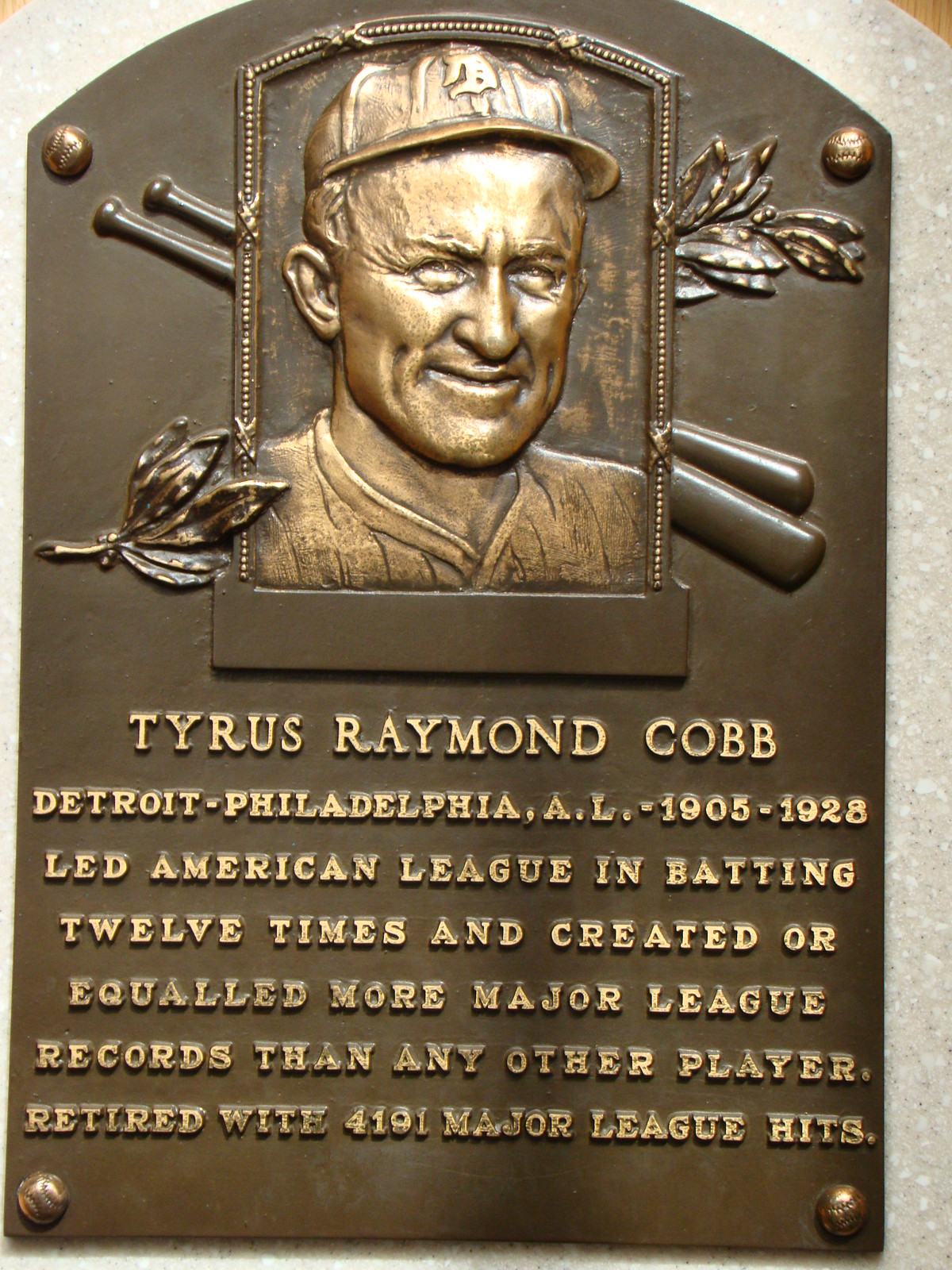**Plaque Description:**

This bronze plaque commemorates the legendary baseball player Tyrus Raymond Cobb, showcasing a detailed bas-relief sculpture of Cobb, adorned with a Detroit Tigers cap. The plaque is prominently brown in color, possibly indicating its bronze material. At the top, the bas-relief image of Ty Cobb is accompanied by crossed baseball bats and a laurel decoration behind the sculpture. Each corner of the plaque features gold baseballs, enhancing the historical elegance. The plaque is set on a marble-like base with a curved top and a rectangular body.

The text on the plaque honors Cobb's illustrious career, stating: "Tyrus Raymond Cobb, Detroit, Philadelphia, A.L., 1905-1928. Led American League in batting 12 times and created or equaled more Major League records than any other player. Retired with 4191 Major League hits." The raised golden letters further emphasize the significance of Cobb's achievements in baseball history.